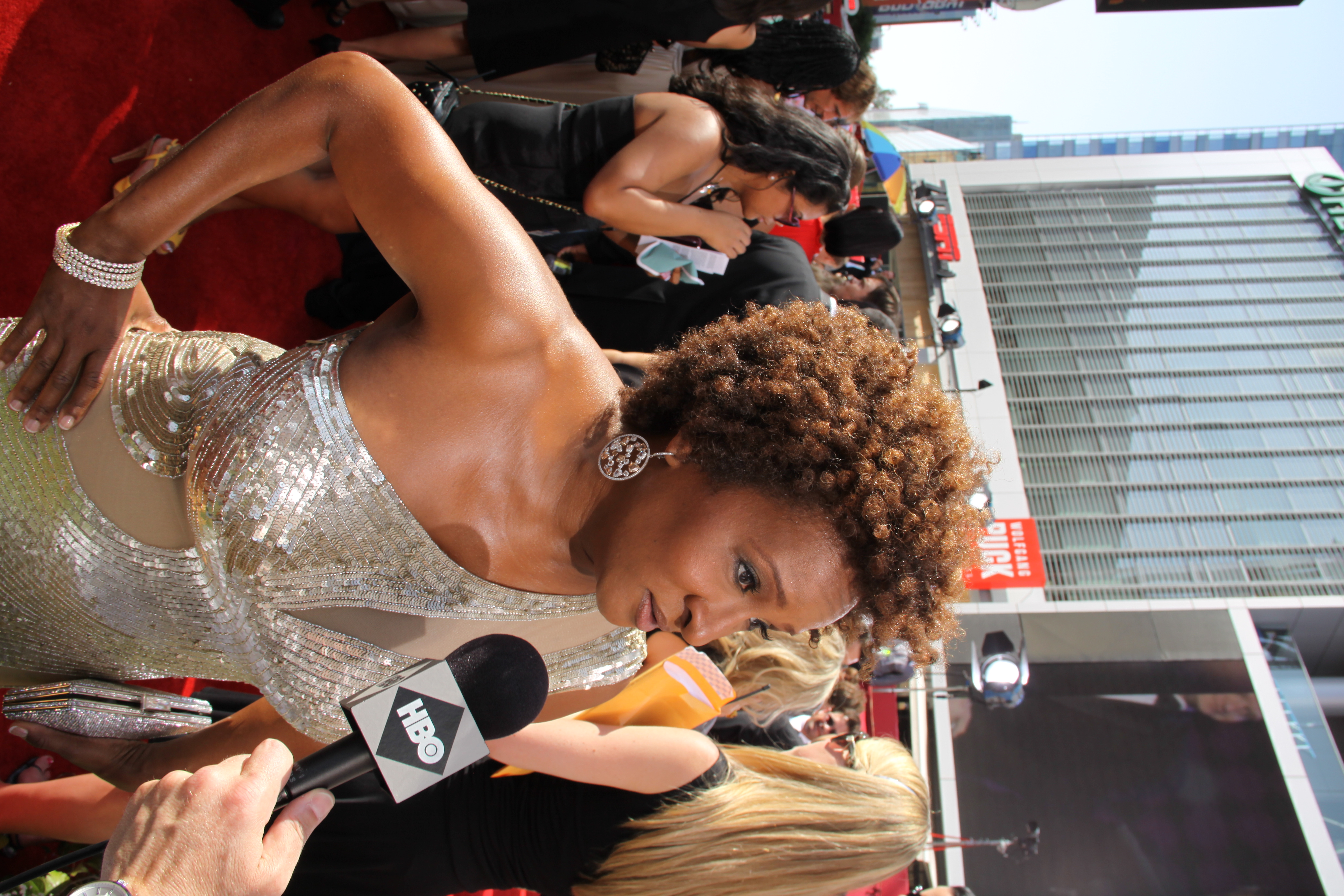The photograph depicts Wanda Sykes at a major award ceremony red carpet event, appearing to be engaged in an interview with HBO. The image, which initially seems rotated 90 degrees, captures Wanda, an African American woman with curly brown hair, confidently standing in an exquisite silver one-strap dress that leaves her right shoulder bare. She accessorizes with silver earrings and a matching clutch in her left hand, while her right hand rests on her hip. A microphone with the HBO logo—black text within a diamond-shaped black square on a gray box—is prominently held by an interviewer in the lower portion of the image. The background reveals other elegantly dressed attendees and a large building, signifying the event’s grandeur. The red carpet beneath them enhances the scene’s opulence and underscores the significance of the occasion.